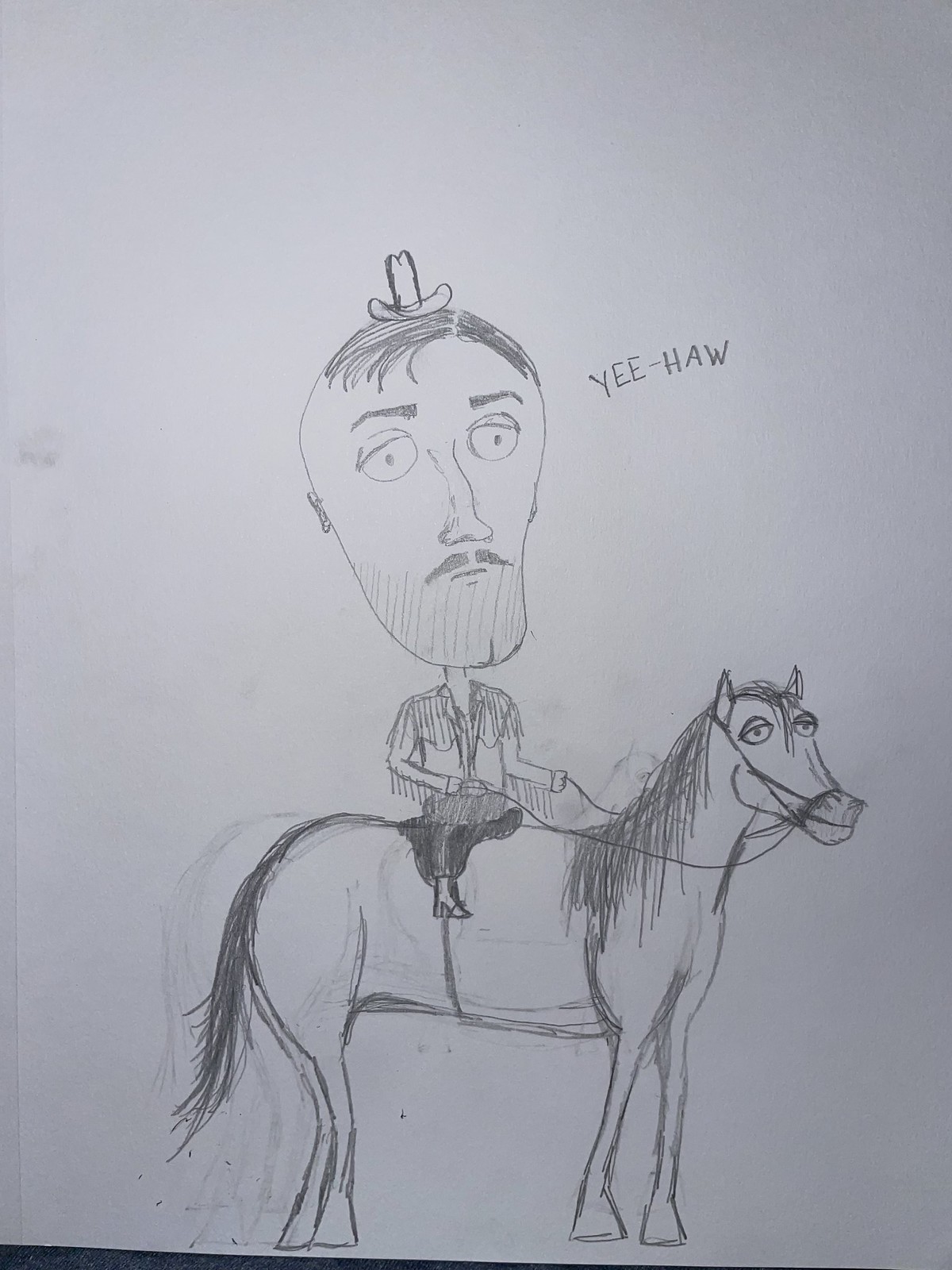The image captures a photograph of a pencil drawing on a white, slightly grey-tinted piece of paper. The sketch, imperfectly erased in parts, portrays a whimsical scene centered around a disproportionate, oversized-headed cowboy riding a horse. The cowboy, with his potato- or upside-down avocado-shaped head, sports a tiny cowboy hat, a mustache, and a faint beard shadow. His large eyes contain just minimal dot details, and his facial expression is unsmiling. Adorning a cowboy outfit, the cowboy wears a long-sleeved button-up shirt with fringes, dark pants, and high-heeled boots. 

Perched on a horse with an unbrushed mane and tail, the saddle and bit details are clearly penciled in. Despite multiple previous attempts visible in the semi-erased lines around the horse’s tail and hooves, the horse is looking to the right with exaggerated big eyes. Floating near the cowboy’s head, the text "YEEHAW," written in all caps, adds a playful touch to this intricately detailed drawing, hinting at a spirited, albeit humorous, western tableau.